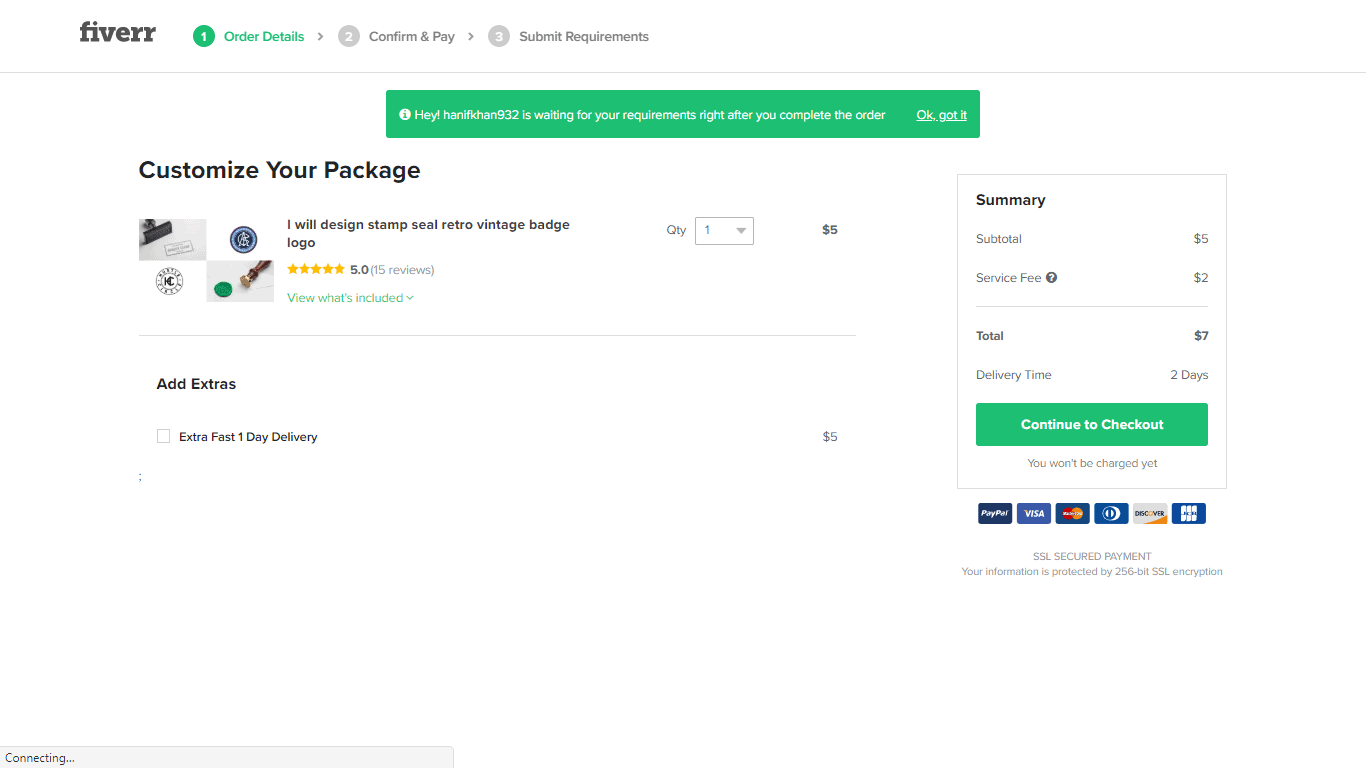In this image from the website Fiverr, we observe several elements laid out methodically against a white background. Starting at the top left corner, the Fiverr brand logo is prominently displayed in bold black text, spelled "Fiverr" with two 'R's. Adjacent to the logo, the webpage illustrates a three-step checkout process. The first step, "Order Details," is highlighted in green to indicate that it is either the current step or has been completed. The subsequent steps are "Confirm and Pay" and "Submit Requirements."

Further down, there is a focused pop-up dialog box containing detailed information about a specific service offering. The offering is titled "Customize Your Package: I will design stamp seal retro vintage badge logo." The cost of this service is listed as $5, accompanied by a $2 service fee, bringing the total to $7. The expected delivery time for this service is mentioned as two days. Below these details, there is a prominent "Continue to Checkout" button.